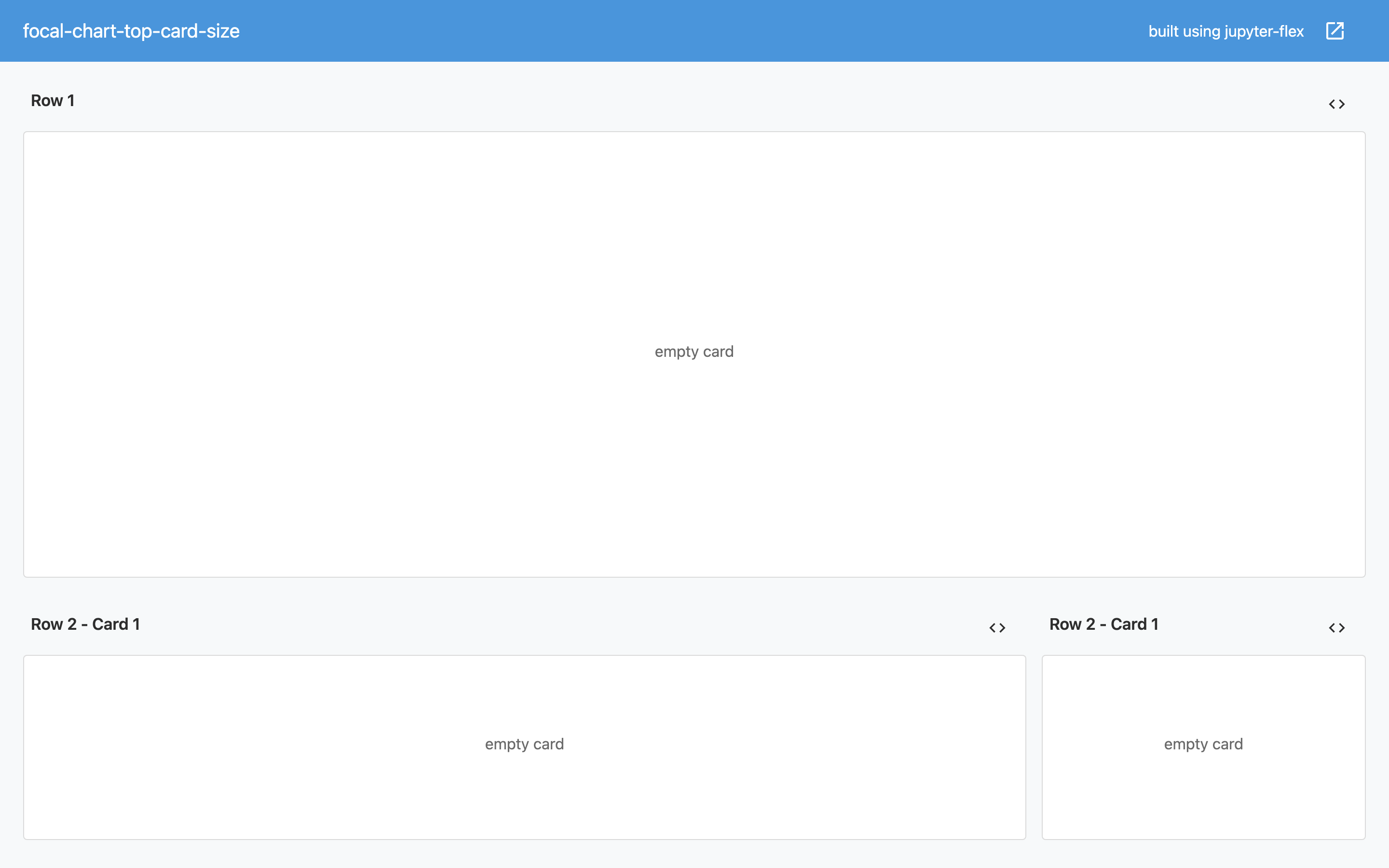This is a detailed screenshot of a settings page within a website or application. 

At the very top, a medium blue rectangular header spans the width of the page. On the left side of the header, white text reads "Focal-Chart-Top-Card-Size". On the right side, white text indicates "Built using Jupyter-Flex", with "Jupyter" carefully spelled out as J-U-P-Y-T-E-R. Adjacent to this text, there's a white square icon featuring a white arrow pointing up and to the right at a 45-degree angle.

Below the header lies the main body of the page, which is set against a light gray background. At the upper left corner of this section, bold text reads "Row 1". Directly across on the upper right, an arrow pointing left sits next to an arrow pointing right.

Beneath this notation is a prominent white rectangle with rounded corners and a faint gray outline. Within the center of this rectangle, medium gray text simply states "empty card" in all lowercase letters.

Continuing down the page, another expanse of light gray background appears. On the left side, bold text notes "Row 2-Card 1". Directly beneath this header is another medium-sized white rectangle similar in design to the first one, also with centralized text reading "empty card".

Above the right-hand side of this second rectangle, another set of left and right arrows is displayed. To the right of this position, there is a smaller card labeled "Row 2-2-Card". It, too, features centralized text stating "empty card" and is flanked on the right side by left and right arrows.

The structured layout and consistent design elements indicate a well-organized settings page, making the user interface navigable and straightforward.